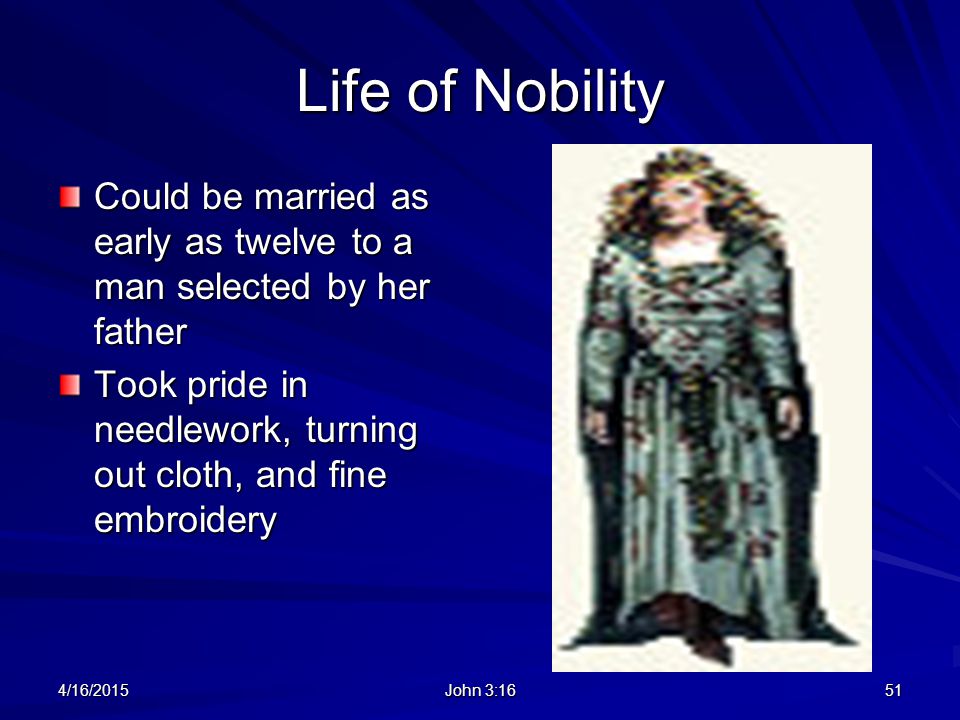The slide titled "Life of Nobility" features a detailed blue background with white text and subtle blue lights emanating from a corner. The text is organized with two main bullet points on the left, highlighting aspects of a noble woman's life. The first point states, "Could be married as early as 12 to a man selected by her father," while the second point reads, "Took pride in needlework, turning out cloth and fine embroidery." On the right side of the slide, there is a pixelated image of a woman dressed in Victorian-era attire—light blue clothing and possibly a crown or headband—against a white background. At the bottom, the date "4-16-2015" is visible on the left, "June 3, 316" is written in the middle, and the number "51" appears on the right.